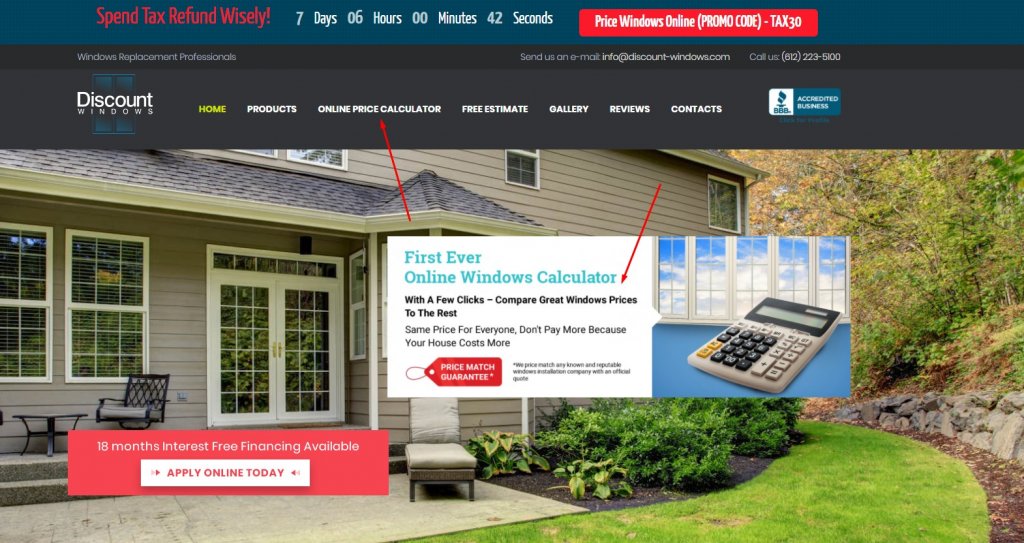The webpage for Discount Windows features a prominent top bar in a greenish-blue hue with striking red text that reads, "Spend Tax Refund Wisely." Accompanying this message is a countdown timer in white text, currently indicating 7 days, 6 hours, 0 minutes, and 42 seconds remaining for a promotional sale. Adjacent to this, a bold red button with the white text, "Price Windows Online" invites visitors to get an estimate, with the promo code "TAX30" noted in parentheses.

Beneath the promotional details, small white text on a black background declares "Windows Replacement Professionals." To the right of this, information for contacting the company is provided: an email address, info@discount-windows.com, and a phone number, possibly 612-223-5100, although it is somewhat unclear.

The main body of the webpage showcases an image of a beautiful home adorned with numerous windows and elegant French doors, suggesting the product offerings. The picture appears to be of the home's rear, featuring a quaint patio area adorned with foliage and lawn chairs, exemplifying the company's quality window replacements in a picturesque setting.